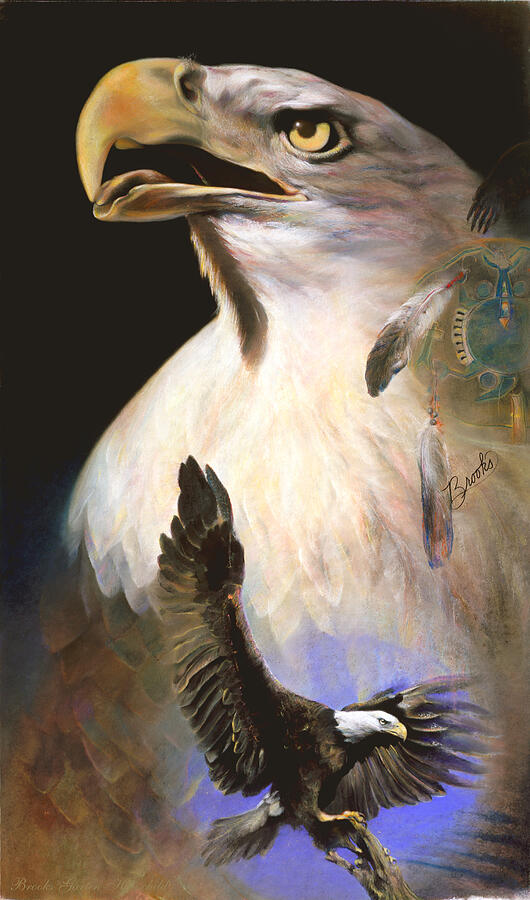This rectangular painting, approximately six inches high and three inches wide, features a detailed depiction of two bald eagles against a black background. Dominating the composition is a close-up of an eagle's head and chest. This majestic eagle, with its white feathers, yellow beak, and golden eye, is positioned towards the upper left with its mouth slightly open, revealing a hint of its tongue. Surrounding this eagle’s head is an intricate arrangement that includes Native American headdress elements and a feather, with the artist's signature, "Brooks," in cursive on the right.

Below this prominent figure, another bald eagle is visible, situated in the lower right-hand corner. This smaller eagle is captured mid-landing on a branch of a dead tree. The landing eagle has its wings outstretched, with the right wing pointing up and the left wing extended to the side. It too has a white head, yellow beak, and long black feathers. This lower eagle is encircled by a bluish-purple light that blends seamlessly with the white feathers of the larger eagle above, creating a cohesive and captivating visual flow.